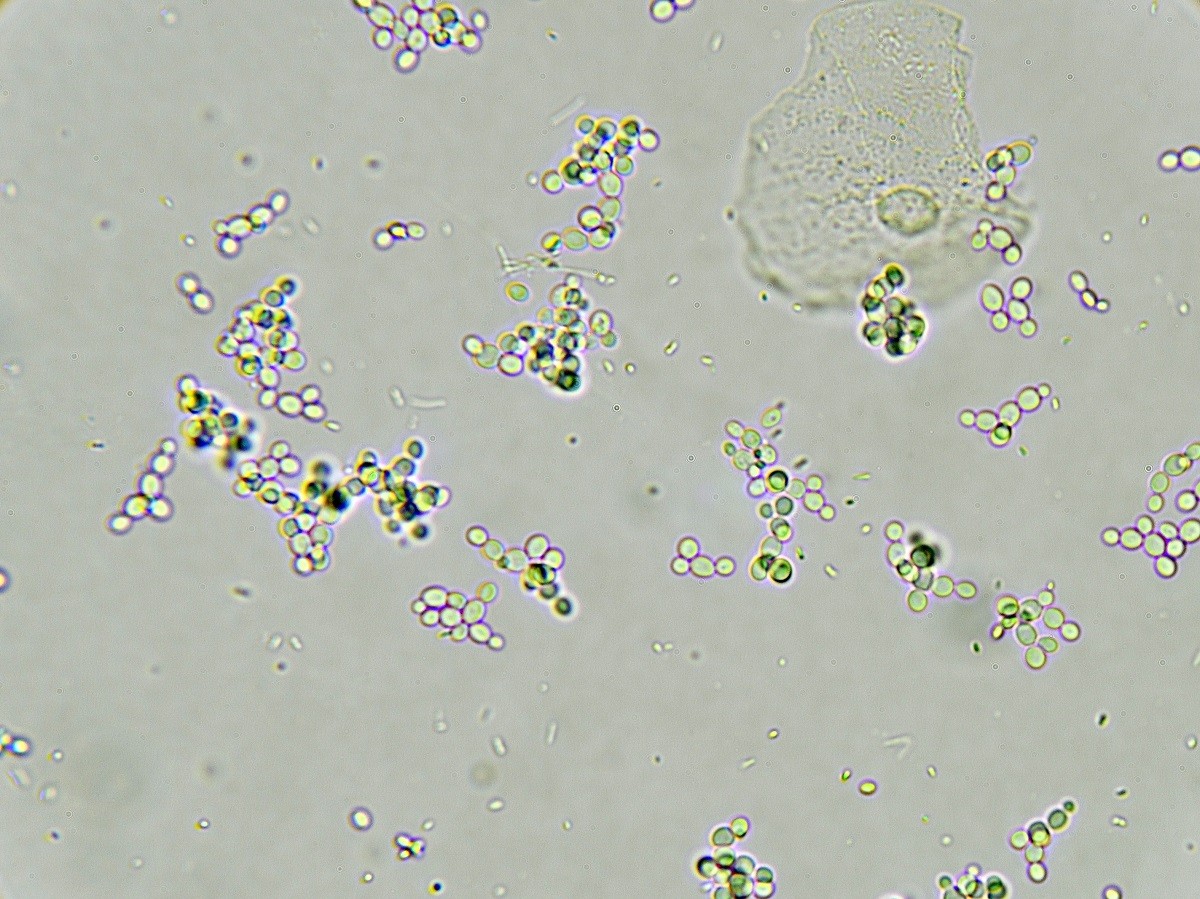This highly magnified microscope photograph features a myriad of microorganisms scattered across a light gray background. The organisms, predominantly green and light green, vary in detail—some exhibiting intriguing purple edges and others appearing more whitish. The image draws immediate attention to a prominent, irregularly shaped transparent mass in the upper left corner, resembling a jellyfish. Encased within this gelatinous blob is a small, oval microorganism outlined in green. Surrounding this central structure are groups of 5 to 12 small dots, ranging in color from cream to dark green, interspersed with tiny light-colored specks. The shapes of the organisms often resemble interconnected circles, suggesting complex formations. This clear, intricate image serves a scientific purpose, primarily inviting observation and study without any guiding text.